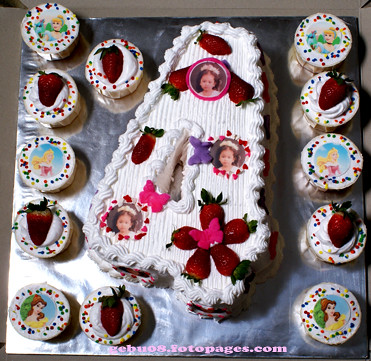The photograph features an intricately designed birthday cake and an assortment of matching cupcakes, all set on a silver foil sheet. The centerpiece is a cake in the shape of the number four, celebrating a Year 4 milestone. The cake is adorned with vertical stripes of white frosting and piped edges, with a large white icing number 4 in the middle. It prominently features edible prints of a little girl, bordered with red and hot pink sprinkles, and a hot pink border at the very top middle. Surrounding the cake are decorative elements, including five strawberries arranged into a floral pattern in the bottom right corner and additional strawberries on the top and sides.

Disney Princess themes are prevalent throughout the display, with edible prints of Cinderella in a blue dress, a princess in a pink dress, and Belle in her iconic yellow gown with brown hair. The cupcakes, twelve in total, encircle the main cake, alternating between designs with white frosting and multicolored sprinkles, and those topped with strawberries, some appearing freshly glistening.

At the very bottom center of the foil sheet, there is a website printed in light pink font: G-E-V-U-O-A dot Y-O-T-O-P-A-G-E-S dot com. The entire arrangement is meticulously designed, reflecting a whimsical and celebratory theme fit for a young child's birthday.